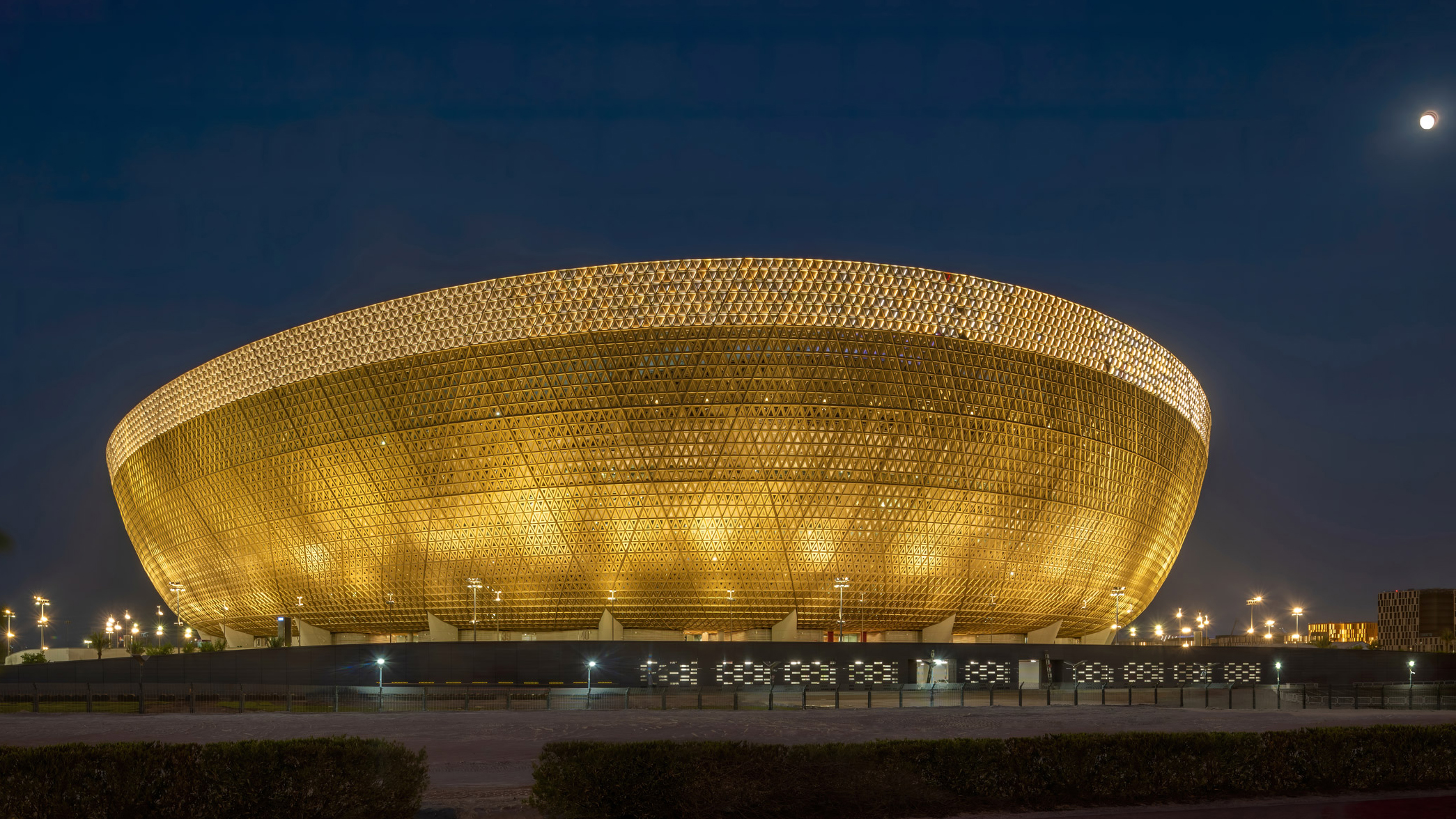The image depicts a horizontally aligned rectangular photograph capturing a large, gold stadium shaped like an upside-down dome or bowl. The stadium exhibits a geometric exterior made up of interconnected triangles and rectangles, giving it a hexagonal pattern overall. This gold structure is illuminated from within at the bottom, casting a glowing yellowish light. The scene appears to be just after dusk, as evidenced by the dark blue evening sky overhead, which exudes a peaceful and serene ambiance. On the right side of the image, a circular white light, possibly the moon, adds to the overall lighting. Below and around the stadium, streetlights are visible along with what seems to be grass and a T-shaped sidewalk leading to a road, although it’s unclear if it’s meant for driving or walking. In the lower section of the image, you can see land, which might include a concrete wall possibly separating the stadium from a parking lot area, but the details are obscured. The stadium's grandeur and the richness of the gold color, combined with the evening setting, lend the image an elegant and luxurious feel.